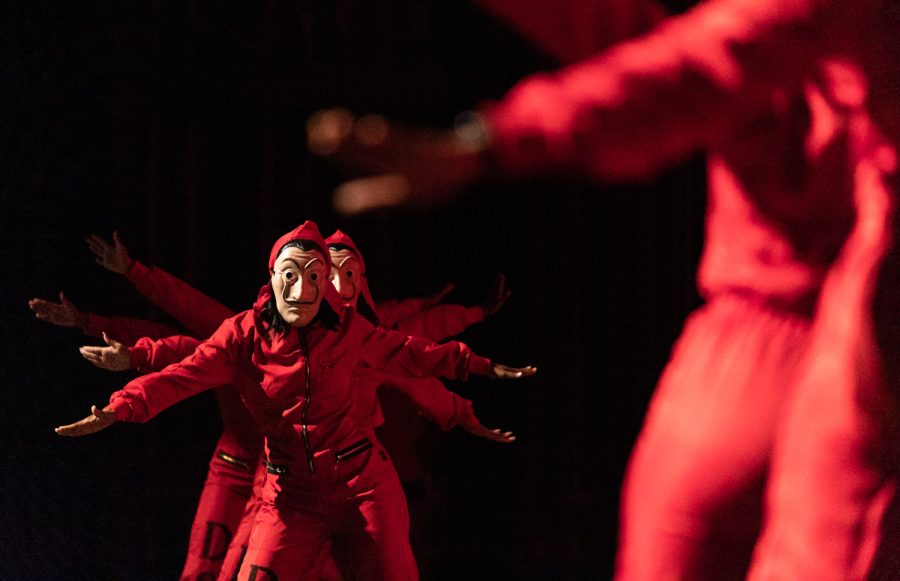The image is a color photograph in landscape orientation, featuring dancers dressed in red jumpsuits with long sleeves and hoods, reminiscent of costumes from the movie "Money Heist." These jumpsuits have black zippers running from the neck to mid-waist and horizontally across the hips, adorned with a black letter "D" on the thigh. The dancers wear plastic masks with big eyes, a prominent mustache extending from under the nose to the eyes, and black wigs, resembling Salvador Dali masks. The backdrop is entirely black, heightening the dramatic effect. In the foreground, a row of dancers stretches their arms outward while facing the viewer, suggesting a moment of synchronized movement, rehearsal, or performance. Additional figures appear on the right side, seen from the shoulders to mid-thigh, with their backs to the camera, adding depth to the composition. The overall style is photographic representationalism realism, capturing the blurred motion and intensity of the dance.